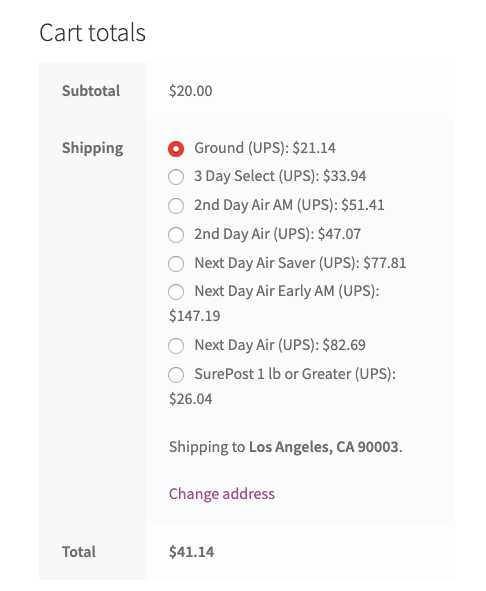The image presents a detailed breakdown of cart totals, with "Cart Totals" at the top left in gray. Below this heading, there is a structured table with two columns: the left column in a slightly darker gray and the right column in a slightly lighter gray.

In the left column, subtitled "Subtotal," "Shipping," and "Total" are displayed in slightly bolded, dark gray text. Corresponding to each row, the right column lists the relevant numerical values:

- Next to "Subtotal," the amount is $20.00.
- Under "Shipping," various options are listed with radio buttons; the selected option is highlighted with a red dot. The highlighted option is "Ground UPS" priced at $21.14. Other listed options include:
  - "Three Day Select UPS - $33.94"
  - "Second Day Air AM UPS - $51.41"
  - "Second Day Air UPS - $47.07"
  - "Next Day Air Saver UPS - $77.81"
  - "Next Day Air Early AM UPS - $147.19"
  - "Next Day Air UPS - $82.69"
  - "Sure Post 1 lb. or Greater UPS - $26.04"

- Additionally, the shipping destination is indicated: "Shipping to Los Angeles, CA 90003," which is accentuated with bold text. Adjacent to this, a purple link labeled "Change Address" appears, providing an option to modify the shipping address.

Finally, the "Total" amount, bolded for emphasis, is displayed as $41.14.